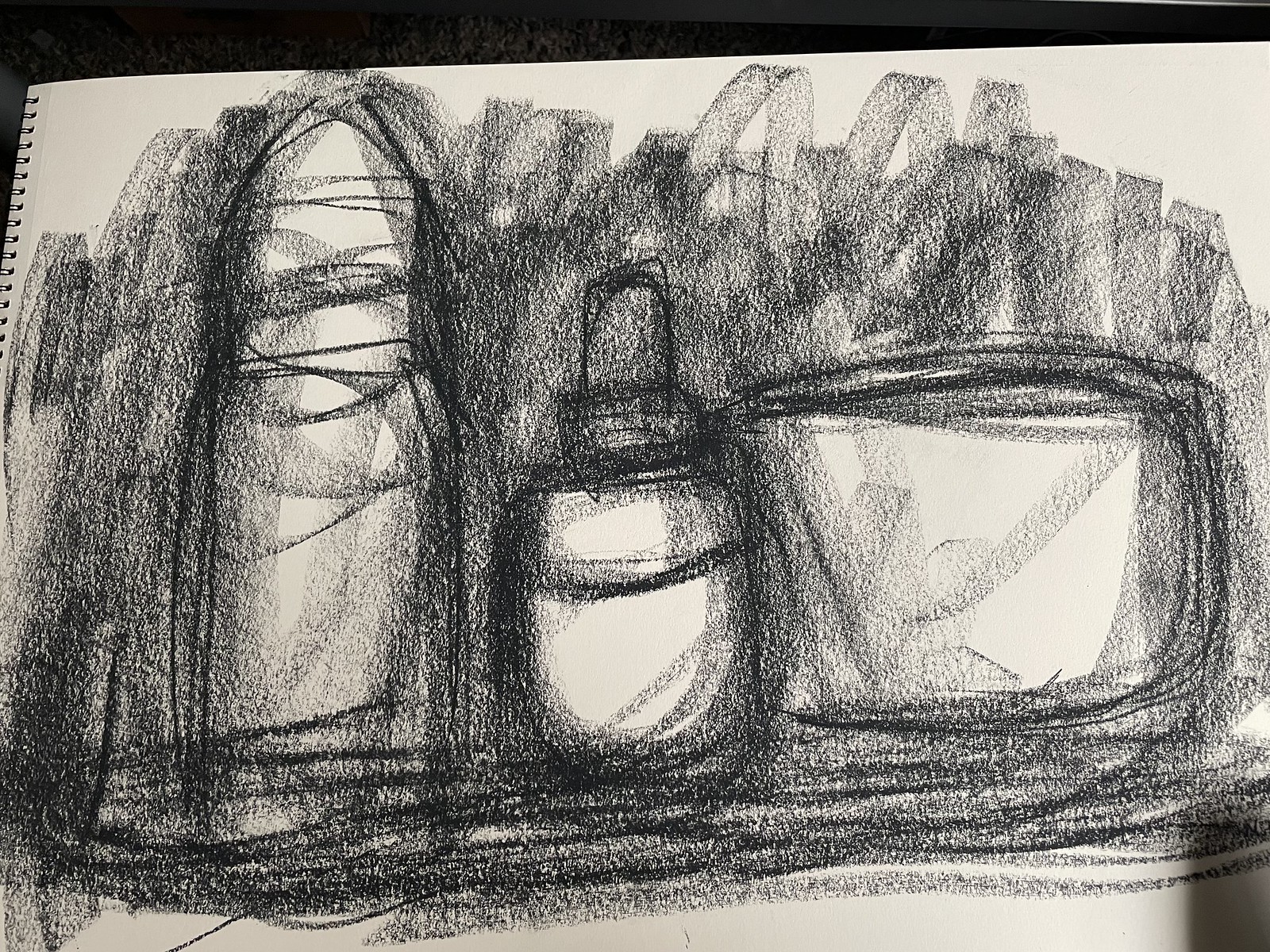This photograph captures a page from a white rectangular sketchbook, identifiable by the visible spiral binding on the left side. The sketch is a loosely drawn, rough graphite pencil illustration, heavily characterized by overlapping lines, and lighter sections indicating highlights or empty spaces within the drawn items. The backdrop under the paper appears to be a black or dark gray carpet flooring. The drawing itself showcases three distinct items: a tall container on the left resembling a thermos flask with a thinner cap, a shorter bottle in the center featuring a dropper, which suggests it could be a type of medicine bottle, and a rectangular object on the right resembling a toiletries bag, potentially housing some items or papers indicated by the shading. The entire composition uses varying shades of graphite and lacks color, enhancing its sketch-like quality.